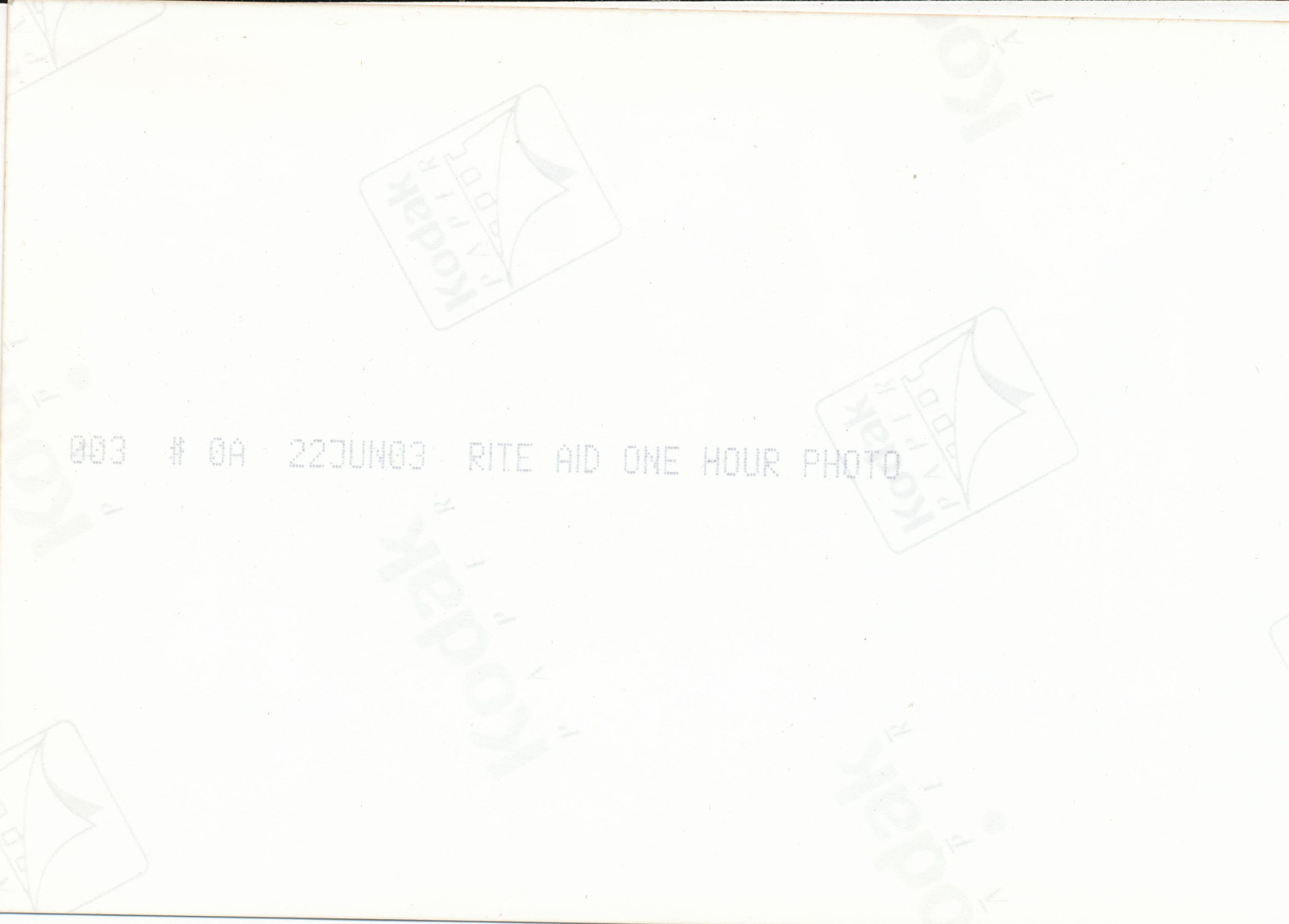The image appears to be a scan of the back of an old, printed photograph. The back side, which is slightly off-white and faded, showcases the Kodak paper watermark repeated across, along with a small emblem of a film strip with a piece of paper emerging from it. In addition, there is faint, light gray text that reads "003 # OA 22 June 03" and "Rite Aid one-hour photo." The original photograph seems to have been photocopied or scanned, and there is a subtle shadow outline hinting at the photograph’s edges, suggesting that it might have been handled or torn at one corner.